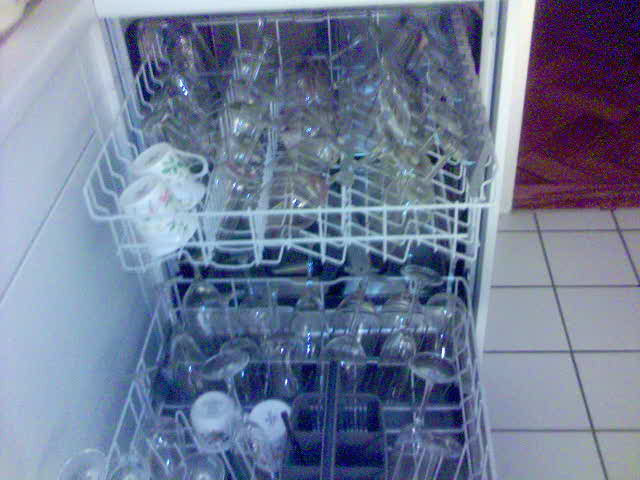The photograph depicts an older, somewhat grainy image of a white dishwasher situated in a kitchen. The dishwasher's door is open, revealing both the upper and lower wire trays fully extended and brimming with glassware. The upper tray holds an assortment of glassware including wine glasses with stems, two white ceramic coffee cups adorned with botanical designs, and some additional glasses without stems. The lower tray is similarly loaded, featuring more footed wine glasses and two matching white ceramic coffee cups. A square plastic silverware holder on the bottom tray is notably empty. The dishwasher is positioned against a backdrop of white cabinet doors to the left and a white tile floor with gray grout that transitions into a beige carpet near an open doorway. A hint of a magenta and orange area rug is just visible in the doorway, adding a splash of color to the scene.